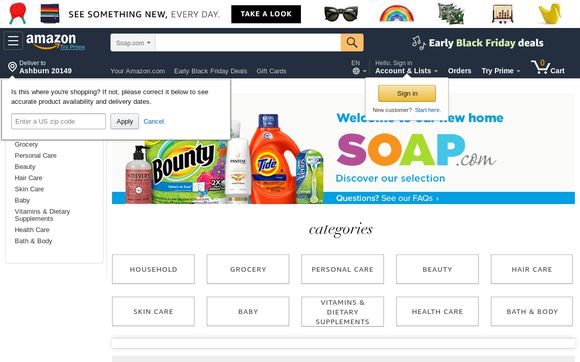The top part of the Amazon website features a prominent black banner with the text, "See something new coming every day." Below this is a black rectangle with the phrase "Take a look" written in white. The image also shows various products including black glasses, a rainbow, green square pillows, a black toy, and a yellow duck. The website's background is blue with the word "Amazon" in white.

The search bar says "soap" in white text, and nearby is the text "early." There is also a green banner with "Black Friday" written on it, followed by a section in white text that includes "Deals" and "Hello, sign in, accounts and list." An orange button, labeled "Sign in," is situated within a black rectangle. Additionally, there is a dropdown indicating the delivery location as Ashburn, VA, 20149. 

Upon clicking this dropdown, the website asks, "Is this where you're shopping? If not, please correct it below to see accurate product availability and delivery dates." There is a white rectangular box with a gray outline where users can enter a US zip code, beside a gray rectangular box with the word "apply" in black. There is also a blue button labeled "cancel."

In the middle of the page, there is a blue section with the text "Welcome, new home, soap.com" and "Discover our selection." Displayed products include Tide, Gillette Razors, Pantene, and Bounty paper towels. The categories section lists items in black text: Household, Grocery, Personal Care, Beauty, Hair Care, Skin Care, Baby, Vitamins and Dietary Supplements, Health Care, and Bath and Body.